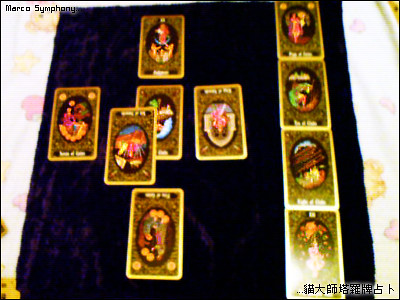The image is relatively small and a bit blurry. In the bottom right corner, there's Japanese text that cannot be translated. In the top left, the phrase "Marco Symphony" is visible. The background features a table draped in a pastel heart-patterned tablecloth, with a black cloth on top. Arranged on this black cloth are several cards, placed in what resembles a tarot card spread, though they don't appear to be actual tarot cards.

On the right-hand side of the black cloth, there is a vertical line of four distinct cards, all connected. The left side of the image, taking up about two-thirds of the space, displays six cards. The arrangement starts with a single card at the bottom row. The middle row has four cards: two are closely spaced, one is somewhat isolated, and another is diagonally positioned over part of a nearby card. The top row features one more card aligned with the bottom card from the three card set. 

Though the card spread mimics the layout of tarot cards, the details and faces of the cards are not legible and some appear to be upside down. All the cards seem to be from the same deck.